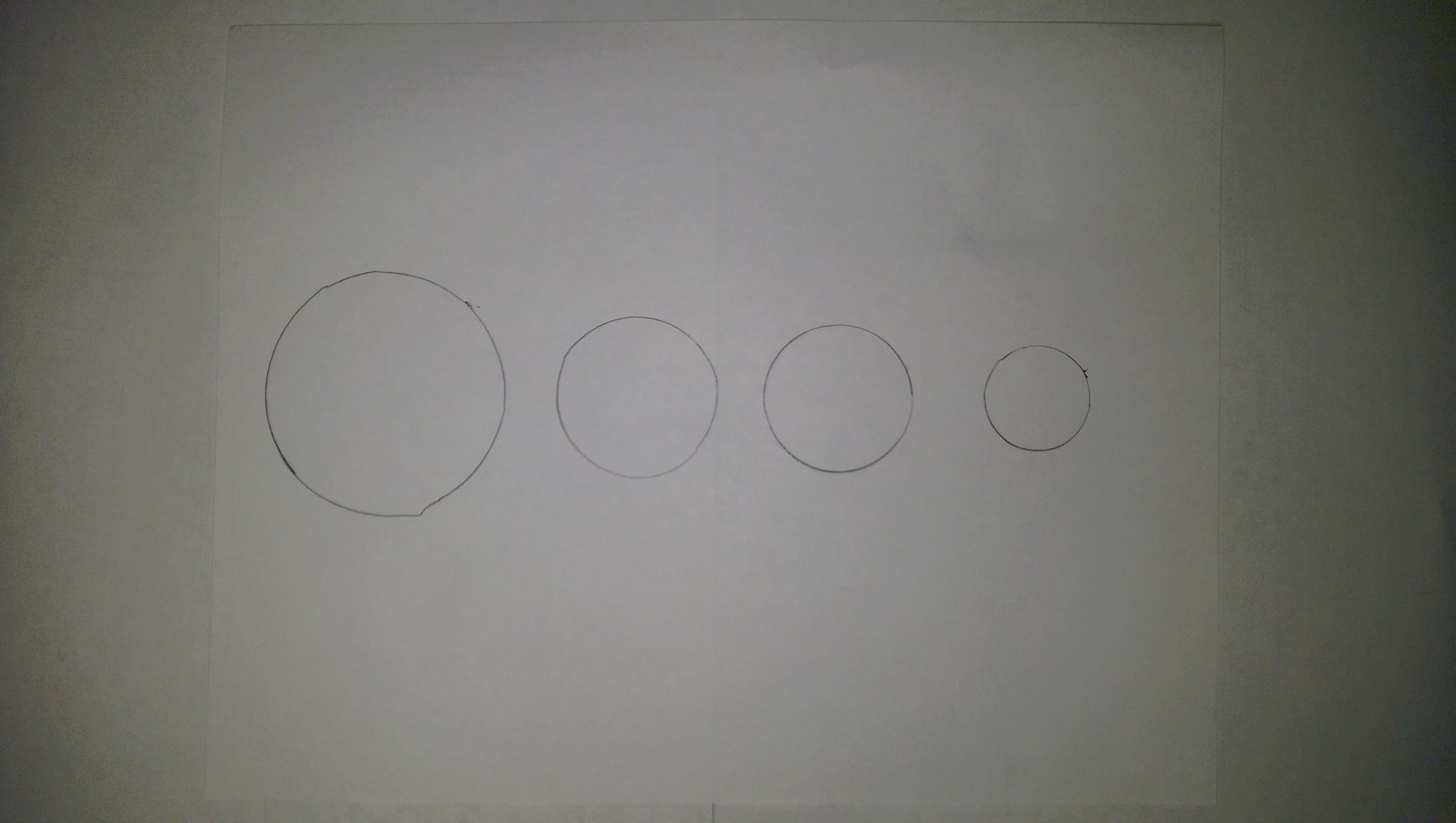In this dimly lit image, we see an unlined, standard-sized (8.5 x 11 inches) piece of white printer paper. The background is also white but shadowed, making it challenging to discern whether the paper is affixed to a wall or placed on a table or fridge. On the paper’s top right corner, subtle smudges and indentations are visible, and there’s a faint grayish mark resembling a small tree with a base and a planter.

Hand-drawn with a black pen, four circles adorn the paper in a horizontal sequence from left to right. The first circle, the largest, occupies roughly a third of the page's upper section if the paper were hypothetically divided into thirds. To the right of this prominent circle is a somewhat smaller one, about half its diameter. Another nearly similar-sized circle sits adjacent to this, slightly larger and more accurately drawn. The final, smallest circle is placed further to the right, not maintaining an equal distance from its neighbors.

The overall composition suggests a casual but intentional sketch possibly conveying some abstract or organizational idea, made more intriguing by the shadows and indistinct background.